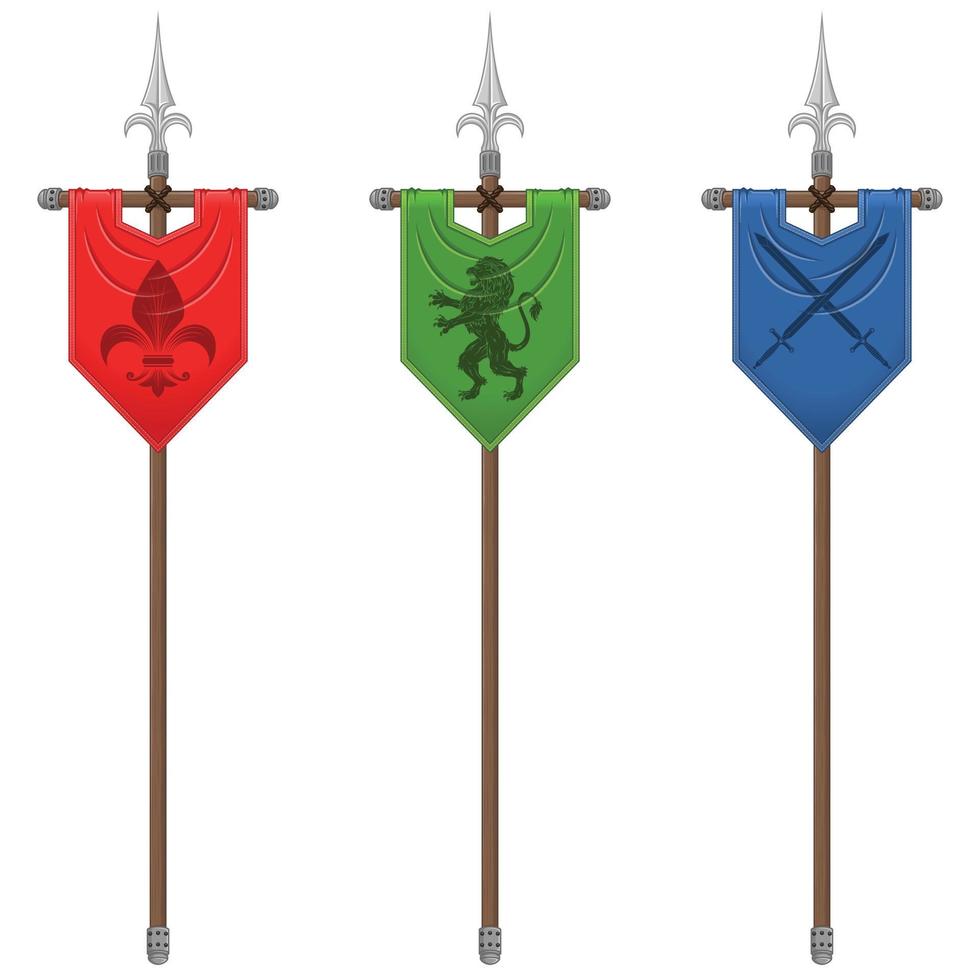The image is a color illustration in portrait orientation, featuring three medieval design standards displayed side by side. Each standard is affixed to a small wooden cross and topped with a silver spearhead flourish, giving them an authentic, medieval appearance. The poles, supported by long, narrow bases, have a distinctive gray knobby end at the bottom and are tied with leather near the top to secure a horizontal cross bar from which the pennants hang.

The first standard, on the left, showcases a red pennant with a blackish-gray fleur-de-lis prominently displayed in the center. This pendant is pointed at the bottom and drapes neatly from its cross bar.

The middle standard is green and features a black lion standing on its hind legs, its tail elevated in an assertive pose. Similarly, it hangs from a cross bar tied with leather near the top of the pole.

The third and final standard is blue, bearing the image of two crossed swords in a light gray or black shade. Like the others, it is pointed at the bottom and suspended from a cross bar at the top of the spear-tipped pole.

Overall, the illustration is detailed and vivid, capturing the essence of medieval heraldry with its consistent and intricately designed standards.